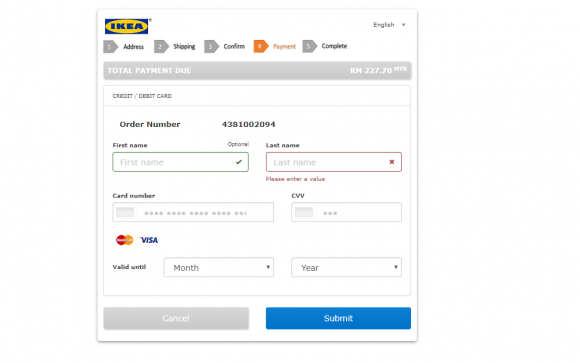The image depicts a website or app interface that is about 20% taller than it is wide, featuring the familiar IKEA logo in blue and gold in the upper left-hand corner. In the upper right-hand corner, black text reads "English" with a down arrow indicating a language selection option.

Below the header, the interface outlines a five-step process for completing a transaction. Each step is represented by a gray arrow with corresponding numbers in white:
1. Address
2. Shipping
3. Confirm
4. Payment (highlighted in orange, indicating the current step)
5. Complete

Directly beneath these steps, a banner spans the width of the image, displaying the total amount due in white capital letters against a gray background: "TOTAL PAYMENT DUE." On the right side of the banner, the amount "RM 227.70" is noted.

Further down, the section prompts for payment method details with the text "Credit/Debit Card" in black, followed by an order number in bold. Fields for entering credit card information are positioned below this text, indicating the final steps to complete the payment.